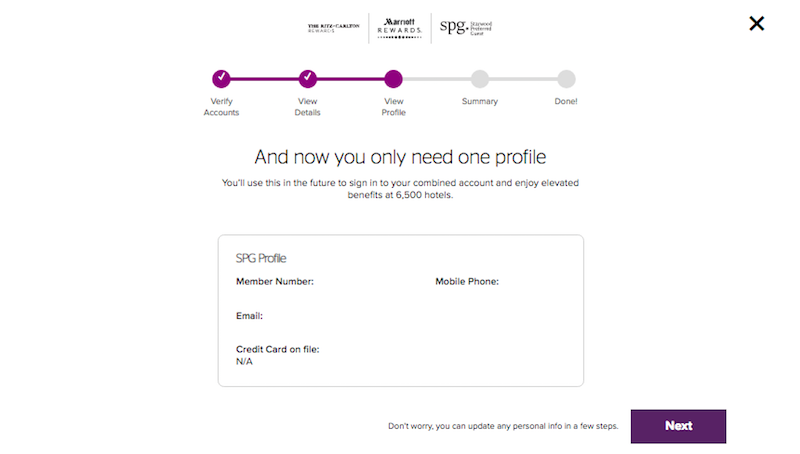**Detailed Caption:**

The image depicts a webpage from the Ritz-Carlton and Marriott Rewards SPG integration portal, characterized by a notably poor resolution. Centrally, there is a streamlined progress tracker comprising five circular icons aligned horizontally. Each icon signifies a step in the profile completion process, starting from the left: "Verify Account," "View Details," "View Profile Summary," and "Done." The "Verify Account" and "View Details" steps have been completed, as indicated by the white check marks within the plum-colored circles. The current step is "View Details," highlighted in plum as well.

Prominently displayed beneath this tracker is the headline in the largest font size: "And now you only need one profile." This statement informs users that moving forward, a single profile will be used to sign into their combined accounts, granting access to elevated benefits across 65,000 hotels.

Directly below the headline is a rectangular information box with a horizontal orientation, containing several fields: "SPG Profile Member Number," "Mobile Phone," "Email," and "Credit Card on File." Presently, all these fields are unpopulated.

Below the information box, on the right side, is a reassuring message: "Don't worry. You can update any personal info in a few steps." Adjacent to this message, on the bottom right corner, is a plum-colored button labeled "Next," which invites users to proceed to the next step.

In the top-right corner of the webpage, there is a white "X" allowing users to close the window. The webpage largely features a color scheme composed of plum, black, white, and gray hues.